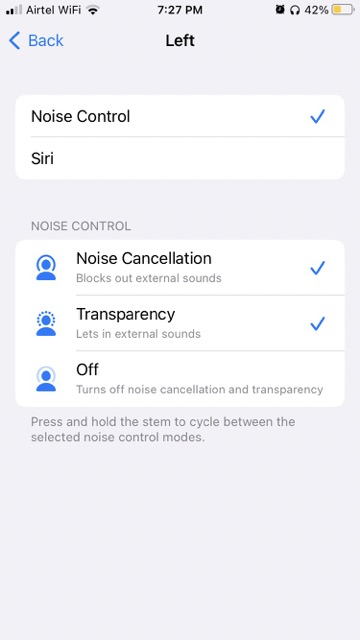Screenshot of a mobile phone interface showcasing the control settings for the left headphone. At the top left corner, the network carrier "Airtel" is displayed with two out of four bars of signal strength. Adjacent to it are the Wi-Fi signal strength, showing two out of three bars, and the current time, 7:27 PM. On the top right corner, icons for headphones, an alarm clock, and the battery level, which is at 42%, are visible.

Below this top bar, the screenshot reveals two tabs: one for "Noise Control," which has a blue tick indicating it is enabled, and another for "Siri," which is unticked. The "Noise Control" section offers three options: "Noise Cancellation," "Transparency," and "Off." Instructions are provided to press and hold the stem of the headphone to switch between these noise control modes. This control panel seems to be specifically for the left headphone, enabling the user to toggle between blocking out external sounds or allowing them in for a more transparent listening experience.